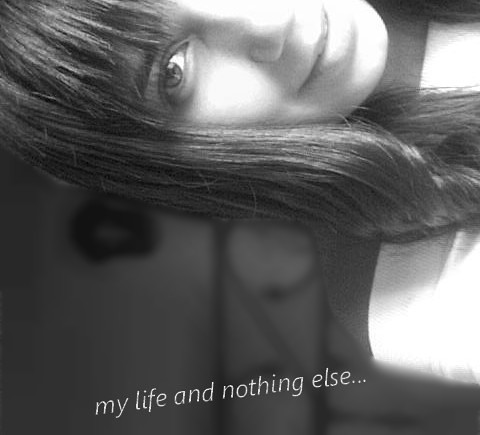The image is a black and white photograph of a woman with pale skin and long, straight brown hair featuring bangs on her forehead. Her face is partially illuminated by sunlight, creating a reflective effect on her skin while the rest of the background remains blurry and dark grey. The photograph is rotated 90 degrees anti-clockwise, causing her face to appear sideways. You can only see one eye and half of her face, which shows her giving a playful little smile towards the camera. She's wearing what appears to be a white dress. At the bottom of the image, slightly slanted white text reads, "My life and nothing else."